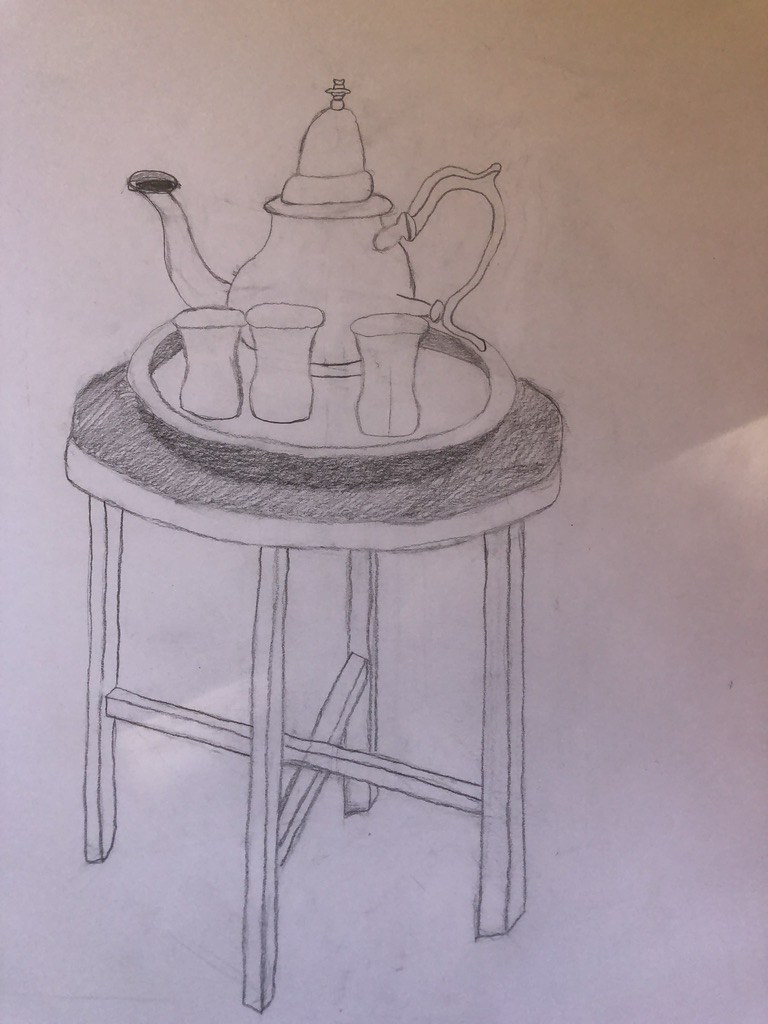The drawing is a simple pencil sketch on a piece of paper that appears lilac gray in the image. It depicts a round stool with four legs, each connected by two crossbars towards the bottom, all illustrated with clean, simple lines. The circular seat of the stool has a slight depth, also drawn with minimalistic lines.

Positioned atop the stool is a circular tray, rendered with a bit of depth and shaded along its sides. The tray holds a teapot that is possibly silver, adorned with ornamental details. The teapot has a graceful handle with a knob, a charmingly bent spout, and a wide, rounded bottom that narrows towards the top, finishing with a lid. Additionally, three glasses sit on the tray, suggesting that the vessel might not be a teapot but a carafe or something similar, given the presence of glasses instead of teacups.